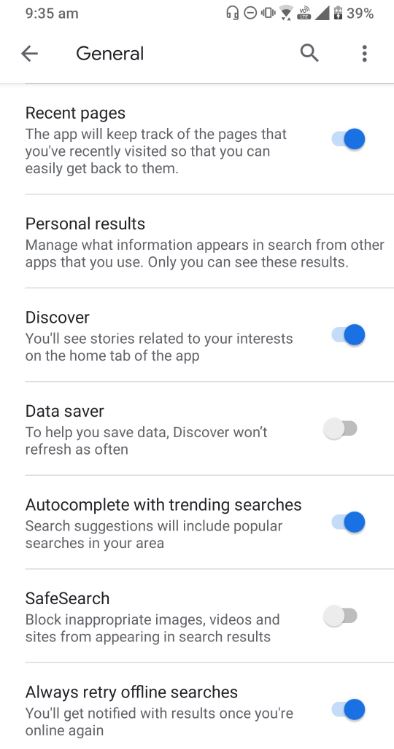The image shows a vertically-oriented screenshot from a cell phone, with dimensions approximately 2.5 times taller than it is wide. 

In the top-left corner, the time is displayed as 9:35 AM. On the top-right corner, there are eight status icons indicating various notifications and statuses, including a battery level at 39%, Wi-Fi signal, and cellular signal strength. 

On the left below the status bar, there is a black left arrow, and to its right, the word "General" is displayed. On the right side of the same horizontal line, there is a magnifying glass icon followed by three vertical dots.

Beneath this, there is a thin horizontal gray line that separates the header from the main content.

The main content features seven sections, each listed with a title and additional details beneath them, and most with toggle switches:
1. **Recent Pages**: Toggled on, with three lines of descriptive text below.
2. **Personal Results**: No toggle switch, with two lines of descriptive text below.
3. **Discover**: Toggled on, with two lines of descriptive text below.
4. **Data Saver**: Toggled off, with two lines of descriptive text below.
5. **AutoComplete with trending searches**: Toggled on, with two lines of descriptive text below.
6. **Safe Search**: Toggled off, with two lines of descriptive text below.
7. **Always Retry Offline Searches**: Toggled on, with two lines of descriptive text below.

The structured layout and toggles indicate settings configuration options for various functionalities of the device.